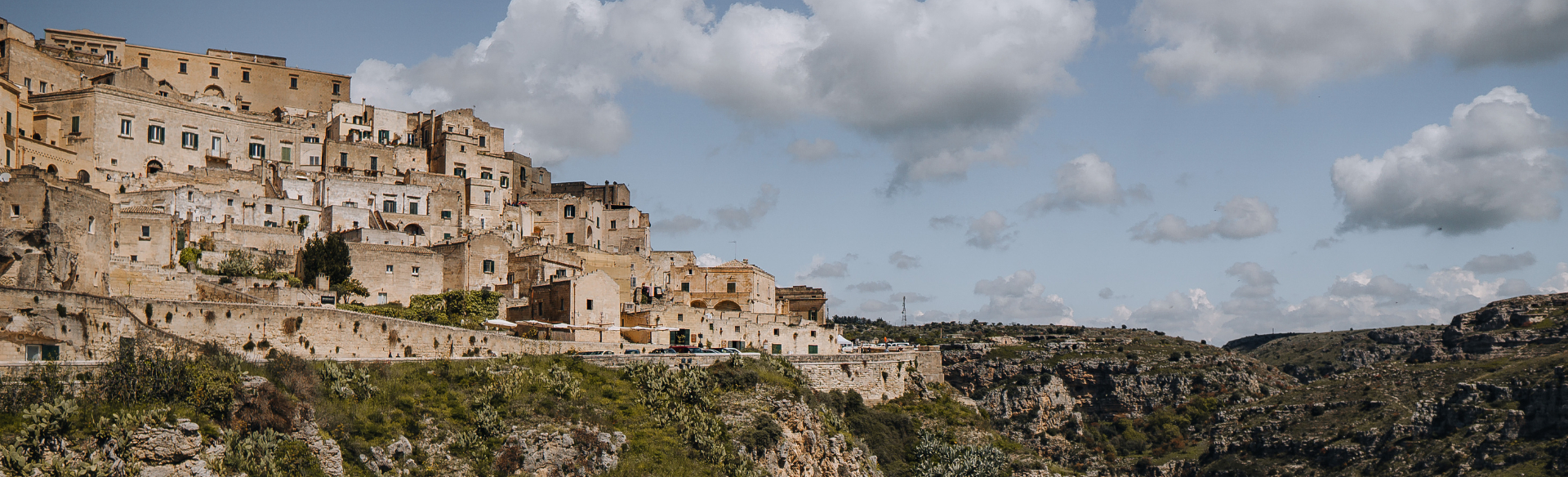This panoramic image captures a picturesque mountainside city, likely in a European country such as Greece or Italy, though it could also be a locale in South America. The photograph showcases a bright, sunny day with a vibrant blue sky dotted with white and slightly gray clouds. The right-hand side of the image features a series of green, rocky hills, while the left-hand side displays a sprawling town built into the mountainside. The buildings, primarily tan, beige, or white, exhibit an old-world charm with their brick and stone facades, many of which appear weathered and worn, with some missing bricks. 

Numerous windows are visible, indicating multi-level structures that create a tiered effect up the hillside. Streets and roadways wind through the town, with several cars visible parked on an overlook, where people can be seen gazing out over the ravine and the lush green valley below. The intricate detailing of the stone architecture and the juxtaposition of natural and man-made structures create a stunning, detailed representation of this serene and historic locale.